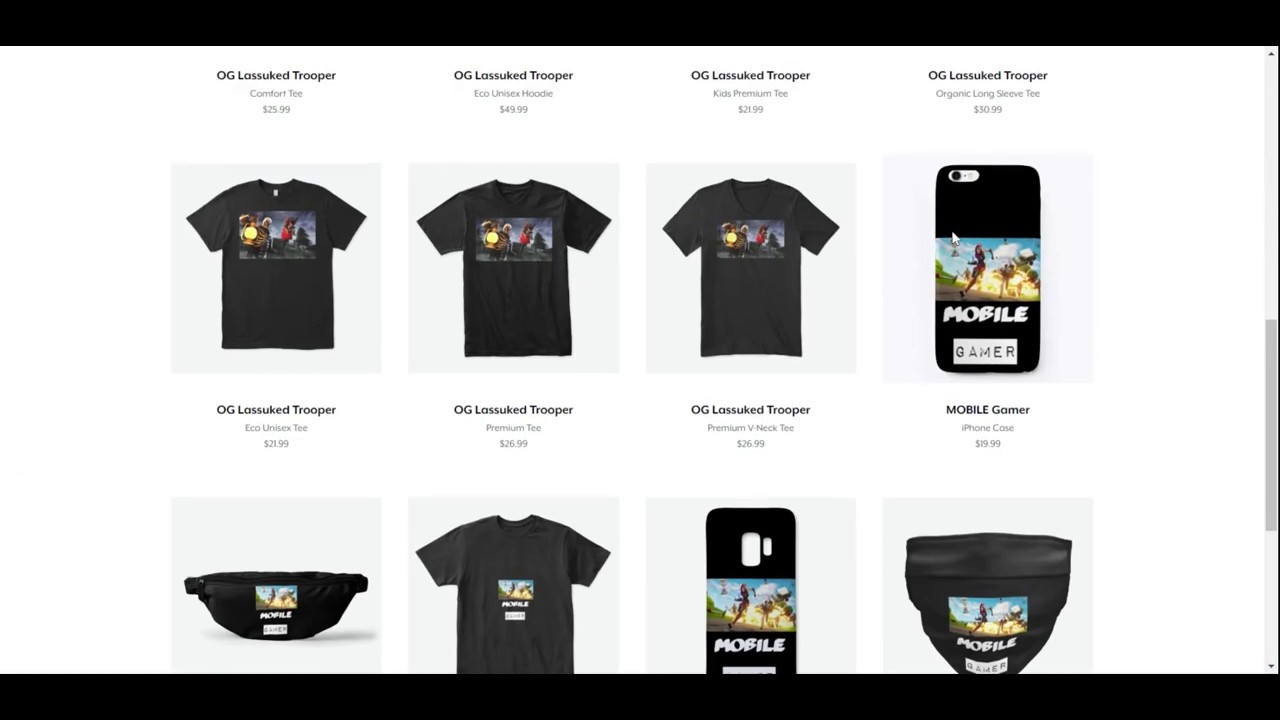This Shopify store appears to specialize in video game merchandise. There are two distinct images featured across various products. The first image, named "OG Lasso Cat Trooper," is displayed on three black t-shirts, which are seemingly unisex standard tees. Due to the small size of the images, details are indistinguishable, but the design appears to involve some form of light or lantern alongside a red object.

The second image, titled "Mobile Gamer," depicts a person either running or jumping away from an explosion, accompanied by the text "Mobile Gamer." This design is printed on a variety of products, including a phone case, a fanny pack, a t-shirt, a differently styled phone case, and what appears to be either a beanie or a face mask. The name of the store isn't visible as the webpage is scrolled halfway down, focusing solely on displaying these products.